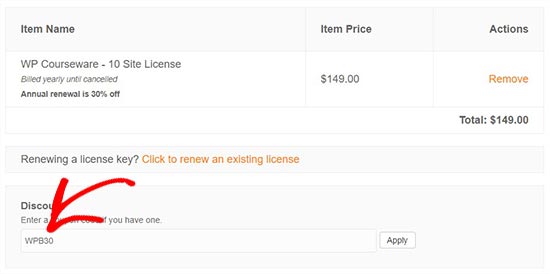The image displays a page formatted as an invoice in the form of a table. At the top of the table, three columns are labeled: "Item Name," "Item Price," and "Actions." 

- **Item Name Column:** Contains "WP Courseware, 10 Site License," with a note stating that it is billed yearly until canceled and that there's a 30% discount on the annual renewal.
- **Item Price Column:** Indicates a price of $149.
- **Actions Column:** Features the option to "Remove" the item, presented as a clickable link in orange.

Below the table, the total price is displayed as $149, and there is a prompt to renew a license key, with "Click to renew an existing license" highlighted in orange as a link similar to the "Remove" option.

Further down the page, there is a box to enter a discount code. A red arrow is drawn, pointing specifically at the box, with the discount code "WP830" indicated nearby. Below the discount box, there is some handwritten text stating "Enter a blank blank blank you have one," though the arrow partially crosses over it, making it somewhat unclear. An "Apply" button is positioned next to the discount code box.

Overall, the screen is neatly organized, providing clear instructions and interactive elements for managing the invoice and potential discounts.